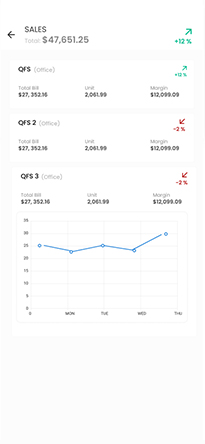The image depicts a data visualization displayed on a white background with various text and numerical data. At the very top of the display, the word "Sales" appears in dark gray text, followed by the term "Total" in a lighter gray shade. Below this, in dark gray, the total sales figure of "$47,651.25" is prominently shown. To the far right, an increase of "12%" is indicated in blue text, accompanied by an upward arrow.

Beneath this section, a white banner presents "QFS (office)" in dark gray, with "office" in light gray. Directly underneath, the total amount "$27,352.16" is listed in dark gray. Some additional data, which appears blurred and unreadable, follow this figure. The pattern repeats with "QFS2 (office)" in dark gray and light gray, respectively, displaying the same amount of "$27,352.16" in dark gray. Likewise, "QFS3 (office)" follows the same format, listing the figure "$27,352.16".

Towards the bottom of the image, a graph is displayed, featuring both vertical and horizontal axes labeled with variables in dark gray. The data points and trends on the graph are illustrated in light blue ink.